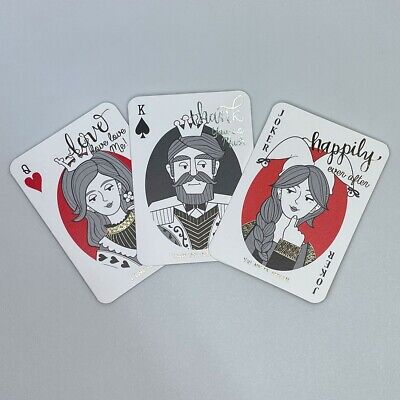In the image, there are three playing cards fanned out against a gray background. The foremost card is a Joker card, prominently featuring an illustration of a woman with gray hair tied into a ponytail, wearing a white jester hat. The card has a handwritten script letter font and the phrase "happily ever after." It also has a red circular border around the figure.

The middle card, slightly to the back on the right side, is the King of Spades. It displays a drawing of a man with a beard, mustache, gray hair, thick eyebrows, and a crown. The card has a black spade symbol and silver foiled text that reads "King" and "Thank you."

The third card, positioned to the left and the furthest back, is the Queen of Hearts. This card features a woman with long, flowing gray hair and a white crown on her head. The card bears a red heart symbol and the repeated inscription "Love, love, love me." Both the Queen and Joker cards are in a red circular border, while the King card has a gray border. The cards are arranged in a gentle curve, suggesting a promotional deck.